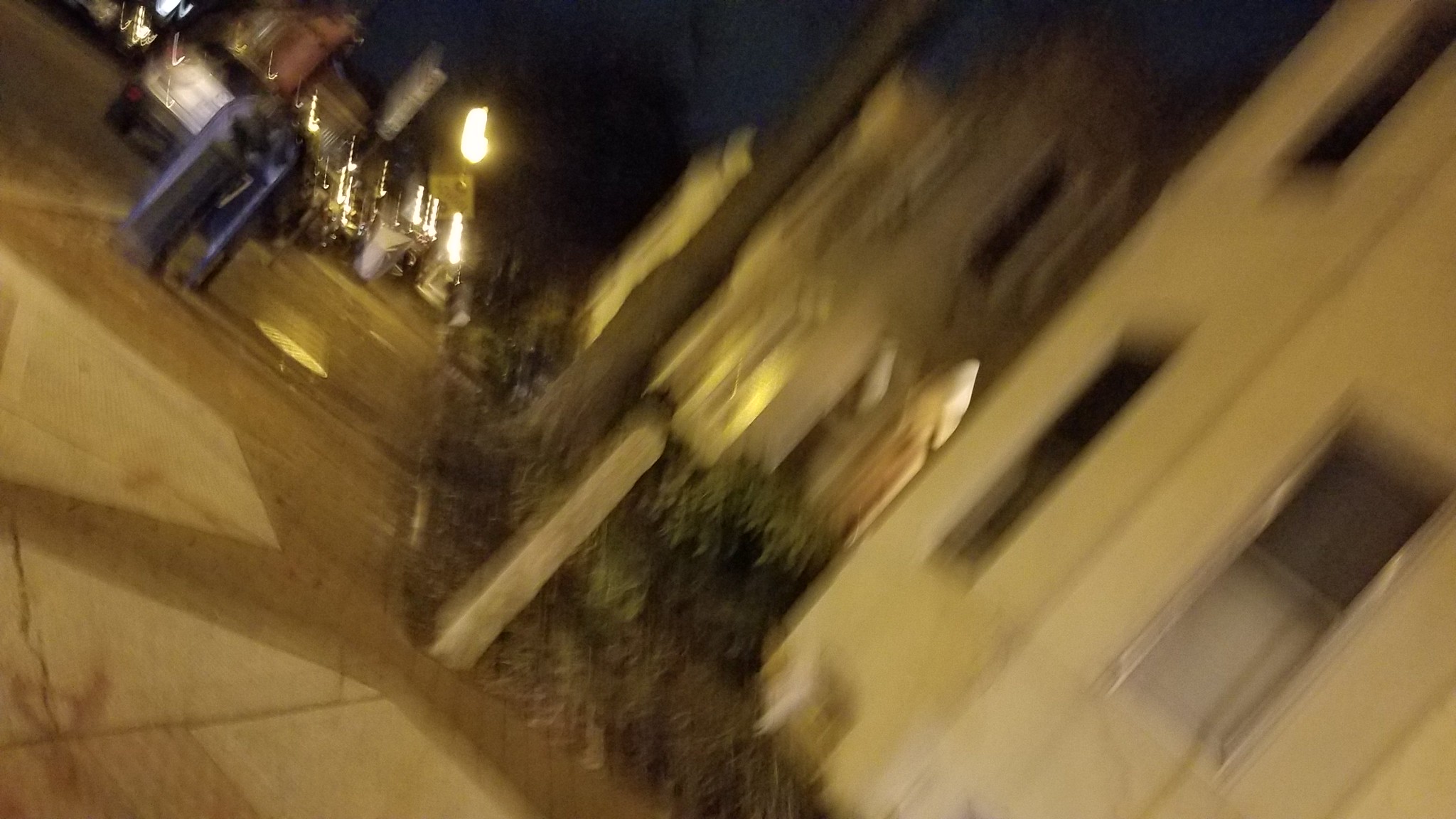In this blurry and tilted nighttime photograph, a city sidewalk scene is captured, likely while the photographer was in motion. The top left of the image reveals a few parked vehicles along the sidewalk, including what appears to be a silver SUV. A hazy streetlight is faintly visible in the same area. The right side of the photograph displays three buildings; the foremost building is white with three elongated, closed windows. Scattered along the sidewalk are black parking meters. Despite the urban setting, no distinguishable people can be identified in the image, and there is no text present. The overall mood evokes a sense of hurried movement through a quiet city street at night.